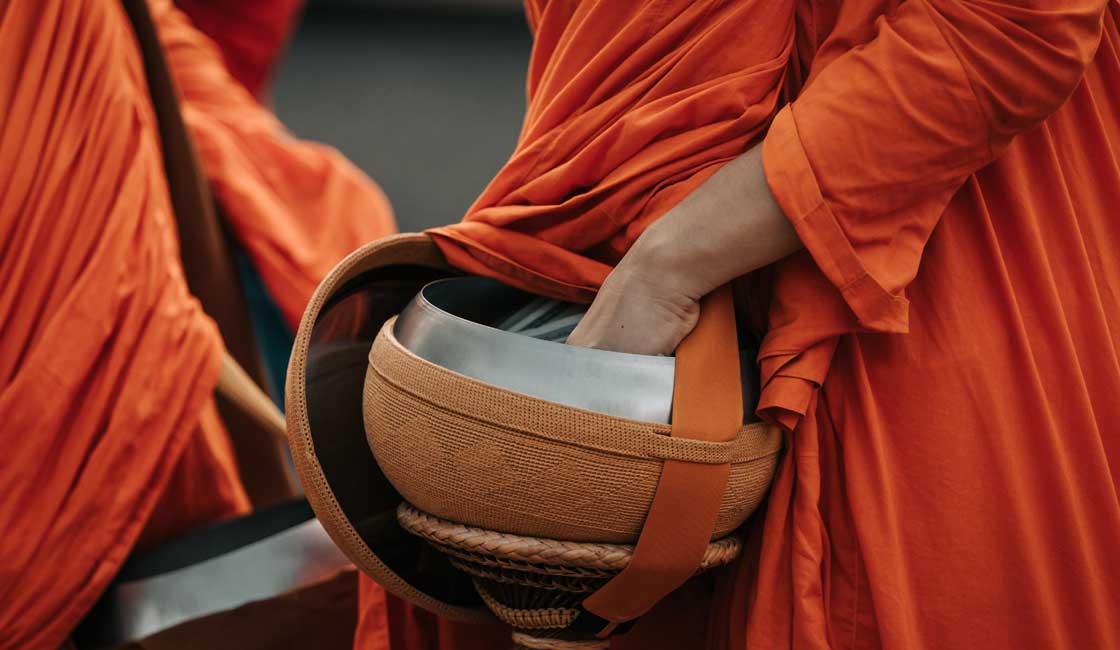In this artistic close-up photograph, we see a detailed scene from the waist down, featuring individuals cloaked in flowing, bright orange ceremonial robes. The central focus is a hand reaching into an urn-like silver bowl, which is nestled inside a dark orange cloth adorned with an ornate diamond pattern, and supported by an orange strap that matches the robes. The bowl seems to have significance, potentially containing items of importance, such as food or ceremonial objects, possibly for a religious or celebratory purpose. The composition also includes part of a chair with a robe draped over it on the left side, suggesting another robed individual facing the opposite direction. The scene evokes a sense of gathering, possibly for soliciting donations or performing a ritual, underscored by the careful, almost reverent manner in which the hand interacts with the bowl. The blurred fingers reaching into the bowl and the matching color palette of the robes, strap, and cloth convey a cohesive, spiritual ambiance.